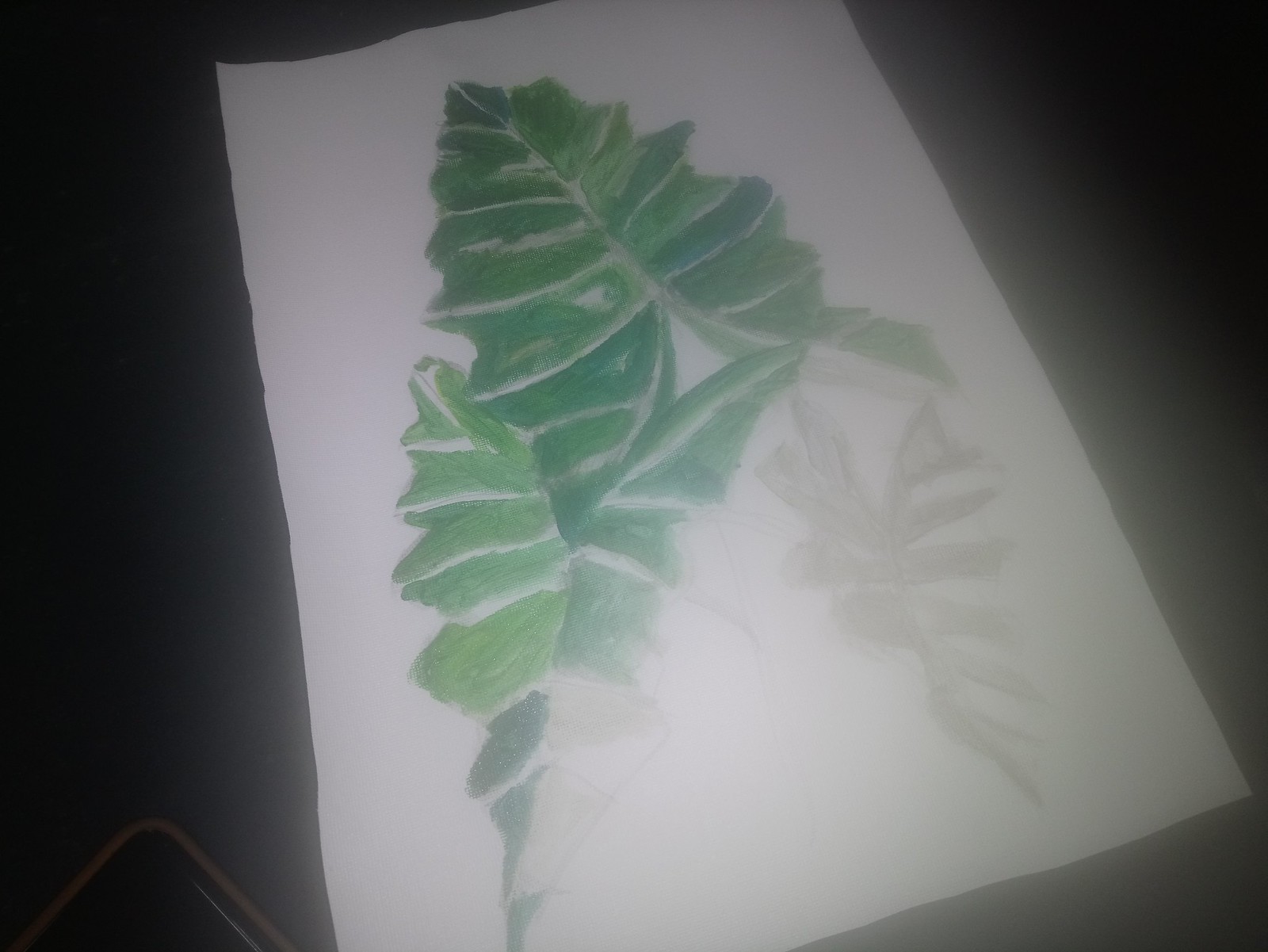This image showcases a meticulously detailed drawing of several leaves on a white sheet of paper. The photograph is taken at an angle, creating a dynamic perspective. The background is a deep black, providing a stark contrast that makes the white paper and green leaves stand out prominently. The leaves themselves are portrayed with a high degree of detail; the veins and serrated edges are clearly defined, emphasizing the organic texture. Among the predominantly green leaves, there is one faint gray leaf, which appears either unfinished or deliberately minimalistic in detail. The composition is focused solely on the leaves and paper, devoid of any other elements or context, highlighting the artistry and intricate design of the leaves.